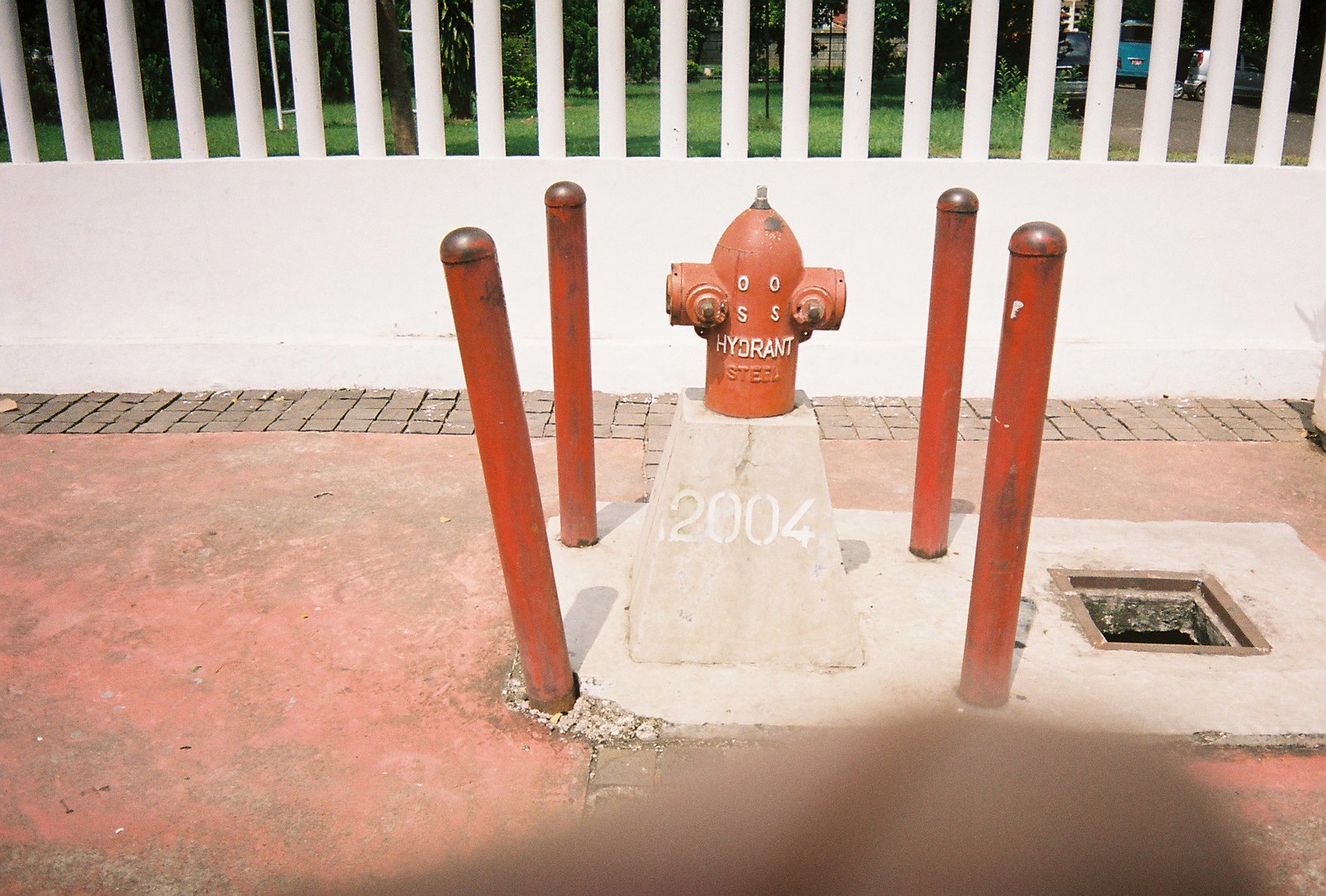The image features a red fire hydrant centrally situated on a weathered, reddish-brown concrete slab that is roughly shaped like a rhombus and bears the inscription "2004." The hydrant itself is old-fashioned with two side connections and is marked with the words "HYDRANT" and "STEEL" in white, along with the alphanumeric sequence "DOSS" or possibly "OOSS." Surrounding the hydrant for protection are four thick, red-painted steel bollards. Adjacent to the hydrant on the right, there is a square hole with a steel frame, revealing a dark void beneath, which appears to lack a cover. The immediate background includes a white vinyl fence about three feet high, with solid panels at the bottom and metal spokes rising above, behind which lies a green yard and a partially visible blue vehicle. The overall scene suggests a residential area captured on a sunny day, with a bit of the photographer’s finger intruding at the bottom edge of the image. The pathway around the hydrant consists of discolored pink concrete with visible dirt and stains, transitioning to a brick walkway further back.